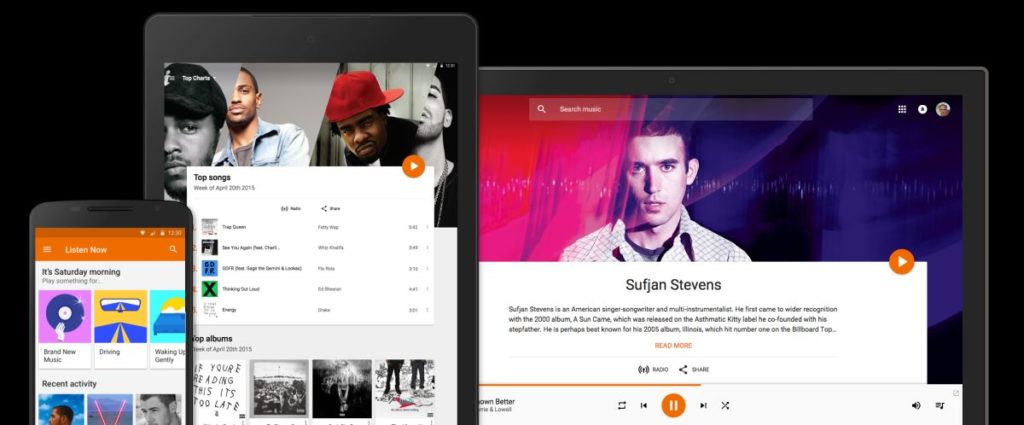The image depicts a dynamic array of devices displaying various media content, all set against a gradient background transitioning from pink on the left to blue and purple on the right. 

On the left side of the image, there's a gray cell phone with a prominent green bar at the top that reads "Listen now." Beneath this, it displays the message "It's Saturday morning, play something for," followed by several options such as "Brand new music," "Driving," and "Walking gently," each accompanied by small icons representing these activities.

Adjacent to the cell phone, slightly to the right, is a gray iPad. The screen showcases an image of four black male music artists, who appear to be rap performers. The artist on the far right resembles Drake, though only part of his face is visible. Above their image, there is a white box labeled "Top Songs," and beneath it, an orange circle with a play arrow. A list of top songs is displayed further down on the screen.

Finally, on the far right of the image, a computer screen features a young white man with short dark hair, wearing a white plaid shirt. He gazes directly at the camera with a neutral expression. At the top of the screen, a search bar reads "search music," while underneath, a white box identifies the man as Sufjan Stevens. The interface below indicates music playback controls with visible icons for stop, fast-forward, and rewind, suggesting that a track by Sufjan Stevens is currently playing.

Each device presents a unique interface related to music playback, highlighting different genres and artists, creating a rich and varied visual narrative.